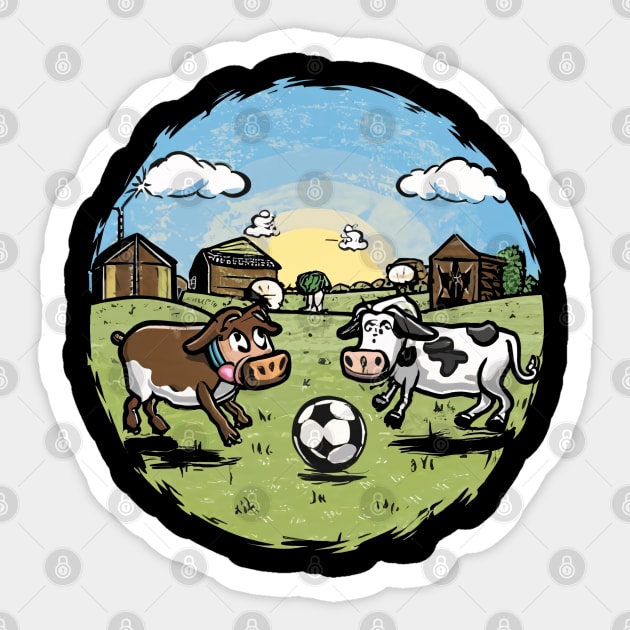This is a detailed digital illustration, possibly a stock image designed to be a sticker, featuring a vibrant and whimsical scene of two cows playing soccer. The sticker has a concentric circular border with a black outer ring and a inner white edge enclosing the main image. Within the circle, a colorful farmland stretches out with green fields, a few small brown sheds (resembling tents) scattered around, and a vivid sunset behind them. 

The sky is painted in shades of blue with white puffy clouds drifting across. The two playful cows dominate the scene; the one on the left is mostly brown with a white underbelly and a bluish collar, while the cow on the right is black and white. They are positioned around a classic white soccer ball with black spots. The landscape and the soccer game blend perfectly with the rural aesthetic, adding a touch of humor and charm. 

Although the illustration is richly detailed with colors like green, yellow, blue, and brown, there is a slightly artificial feel to it, hinting it might be AI-generated. This notion is reinforced by the watermark above the image, which features a lock icon within a gray circle.